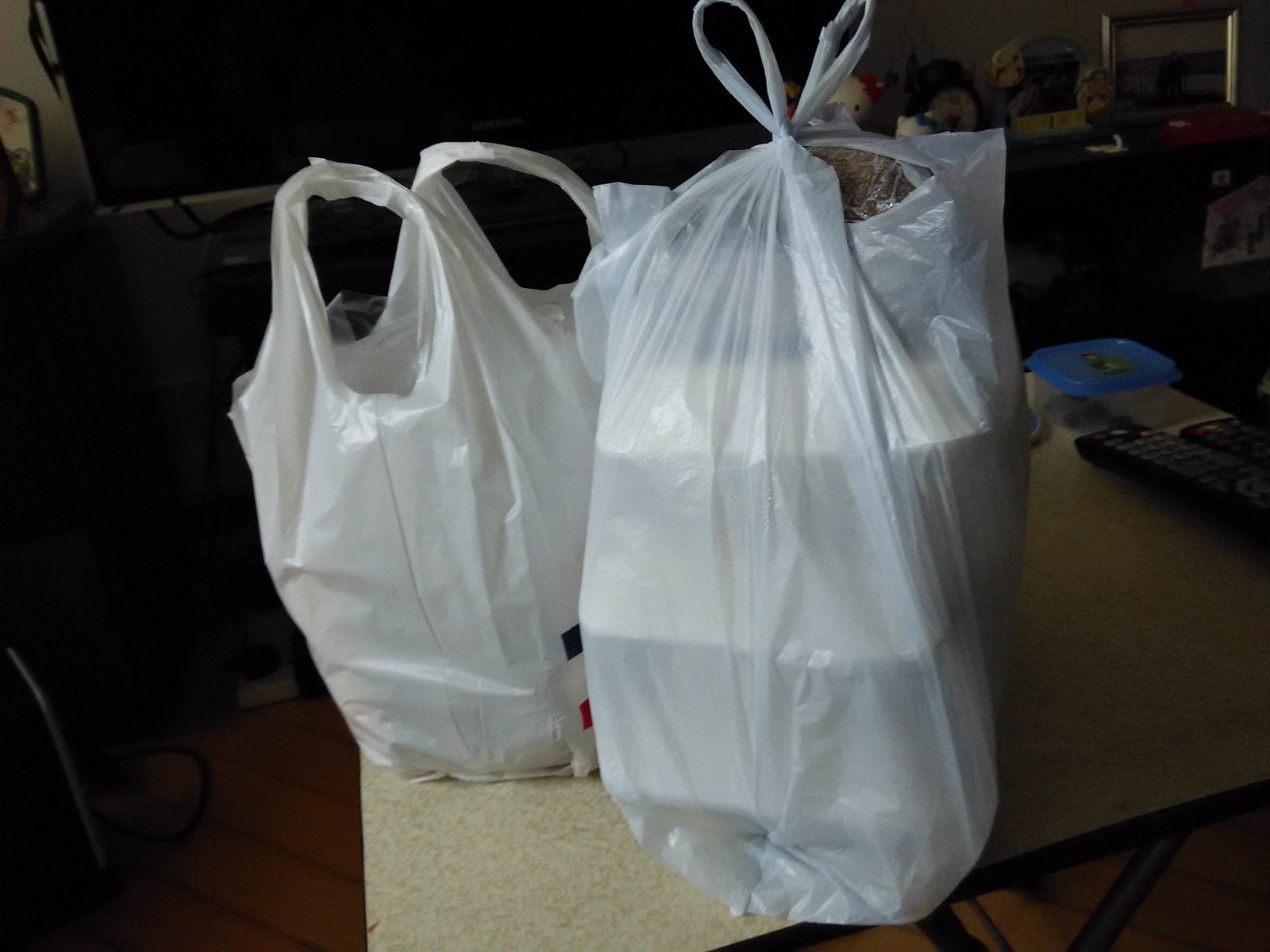In a dimly lit indoor setting, a photograph captures two plastic bags sitting on a light brown tabletop against an almost black background. The right-hand bag is tied at the handles and reveals through its semi-transparent material, four stacked, white Styrofoam take-out containers, likely from a restaurant. To the left, a more opaque white plastic bag stands open with its contents hidden from view. In the top right corner of the image, a blue bowl is faintly visible atop the table. The scene is characterized by its dark ambiance, with the focus squarely on the bags that suggest a recent takeout meal.